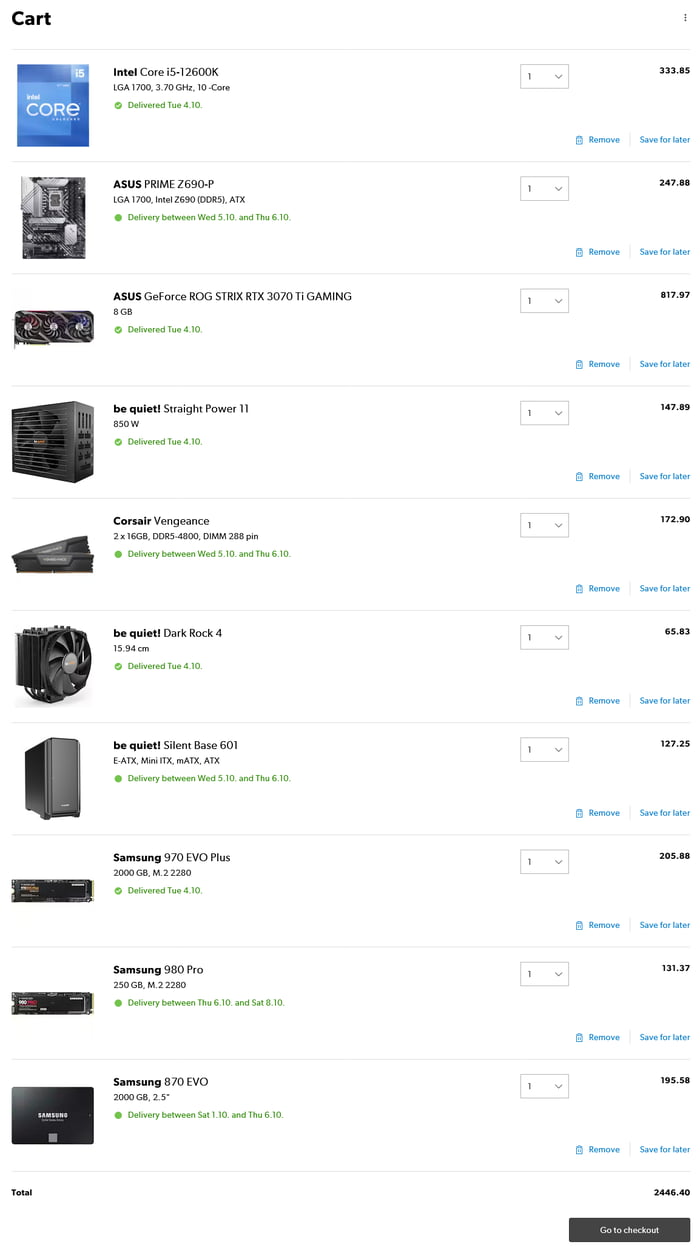**Screenshot of Shopping Cart**

This screenshot captures a shopping cart containing 10 different high-tech items, each accompanied by a thumbnail image on the left. Here's a detailed breakdown of the items:

1. **Intel Core i5 12600K** - Scheduled for delivery on Tuesday, April 10.
2. **Asus Prime Motherboard** - Expected delivery between Wednesday, May 10, and Thursday, June 10.
3. **Asus GeForce ROG Strix RTX 3070 Ti Gaming Graphics Card** - Scheduled for delivery on Tuesday, April 10.
4. **Be Quiet! Straight Power 11 Power Supply** - Scheduled for delivery on Tuesday, April 10.
5. **Corsair Vengeance RAM** - Expected delivery between Wednesday, May 10, and Thursday, June 10.
6. **Be Quiet! Dark Rock 4 CPU Cooler** - Scheduled for delivery on Tuesday, April 10.
7. **Be Quiet! Silent Base 601 Case** - Expected delivery between Wednesday, May 10, and Thursday, June 10.
8. **Samsung 970 EVO Plus SSD** - Scheduled for delivery on Tuesday, April 10.
9. **Samsung 980 Pro SSD** - Expected delivery between Thursday, June 10, and Saturday, August 10.
10. **Samsung 870 EVO SSD** - Expected delivery between Saturday, November 10, and Thursday, June 10.

The total cost for all the items is prominently displayed on the right, amounting to $2,446.40. A black button labeled "Go to Checkout" appears at the bottom of the screenshot, prompting the user to proceed with their purchase.